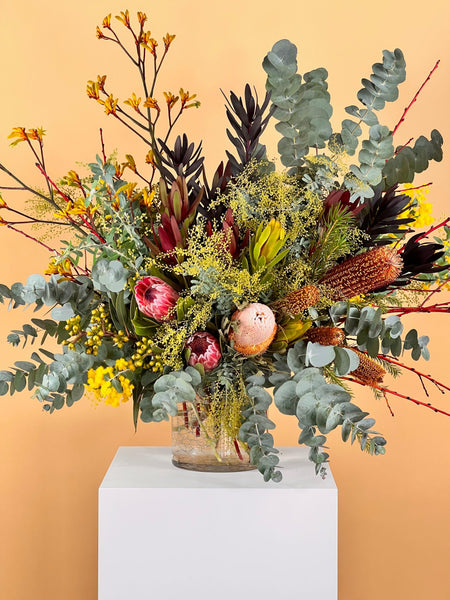The photograph showcases a strikingly beautiful and vibrant floral arrangement. The arrangement is housed in a large, clear glass vase, which sits atop a plain white square stand or pedestal. The backdrop is a soft, peachy orange that enhances the vivid colors of the flowers. The bouquet itself is immense and expansive, overflowing the edges of the stand. The array comprises diverse plant life, including green leafy ferns, various types of yellow flowers—both small clusters and larger single blooms—and a few prominent red flowers. Additionally, there are unique elements resembling fuzzy cattails or brushes, as well as sprigs of tiny flowers. Some stems are bare, adding texture to the assortment. The overall composition is luxuriant with hues of light green, red, peach, yellow, and hints of purplish tones, creating a dynamic and visually captivating display.